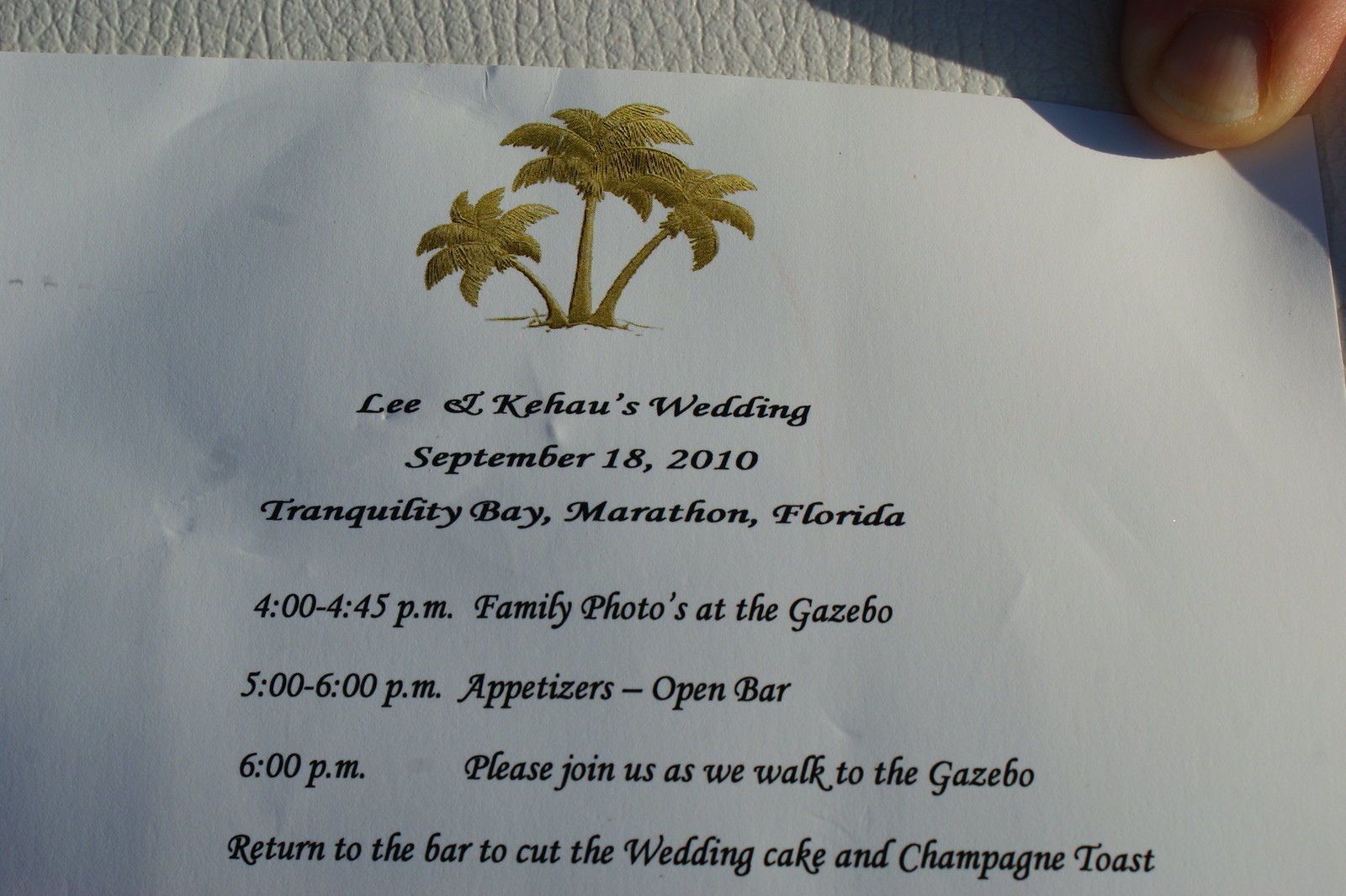In the image, a finger, likely a Caucasian person's index finger, is seen in the top right corner holding down a piece of textured white paper. The paper has a subtly textured background, possibly from a paper towel. At the top center of the paper, there are three palm trees in a gold-green hue: two are leaning outwards to the left and right, while the middle one stands upright. Below the palm trees, bold black text reads "Lee and Kehau's Wedding." The next lines detail the event's specifics: "September 18th, 2010, Tranquility Bay, Marathon, Florida." The schedule follows: "4:00 to 4:45 p.m. Family Photos at the Gazebo," "5:00 to 6:00 p.m. Appetizers, Open Bar," "6:00 p.m. Please Join Us as We Walk to the Gazebo," and finally, "Return to the Bar to Cut the Wedding Cake and Champagne Toast." The entire scene appears to be set on a table, lending an intimate context to this wedding invitation.